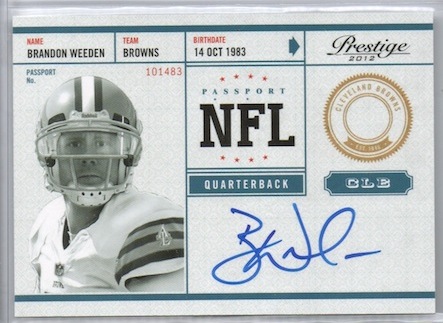The image is of an NFL player's stat card for Brandon Whedon against a white background. The card, which resembles a passport, includes a grayscale photograph of Whedon, capturing him from just above his helmet to just below his chest. He is depicted looking intensely at the camera, wearing a helmet and a short-sleeved jersey with sleeve stripes. The card incorporates colors predominantly in black, white, gray, with accents of red, blue, and gold.

Key details on the card include:
- **Name**: Brandon Whedon, displayed in red and black capital letters.
- **Team**: Browns, indicated below his name in black capital letters.
- **Passport Number**: 101-483, printed in red above the photo.
- **Birth Date**: 14 October 1983, mentioned beneath the team name.
- **Prestige**: 2012, accompanied by a right-pointing arrow.
- **Passport NFL Quarterback** title, positioned next to a gold circular seal that is difficult to read.
- **Signature**: Appearing in bright blue marker, likely a printed feature.

Additional text includes "CLE" and possibly "quarterback" near the seal, again reinforcing his association with the Cleveland Browns. The style and additional adornments suggest this card might be a piece of sports memorabilia, with the signature being part of the card's design rather than a personal autograph.